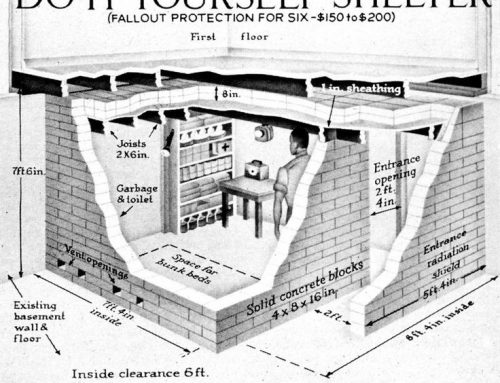This detailed black and white diagram, likely from an old publication or advertisement related to World War I or II, is a blueprint for a do-it-yourself fallout shelter designed to fit within an existing basement. The shelter is labeled "Fallout Protection for 6, $150 to $200" and features a cut-away view revealing the interior layout and construction specifics. The shelter includes brick walls, a solid concrete block entrance opening measuring two feet four inches, and an entrance radiation shield of five feet four inches. The shelter's inside clearance is six feet with a total height of seven feet six inches. Key components are clearly labeled: the first floor, existing basement wall and floor, and joists measuring two to six inches. Inside, a person is seen standing next to a large shelf stocked with noticeable items such as a first aid kit. There is a cabinet for garbage and a toilet, and a designated space for bunk beds outlined with dotted lines. The diagram emphasizes the practical, survival-oriented design, complete with detailed measurements and layout annotations to guide construction.